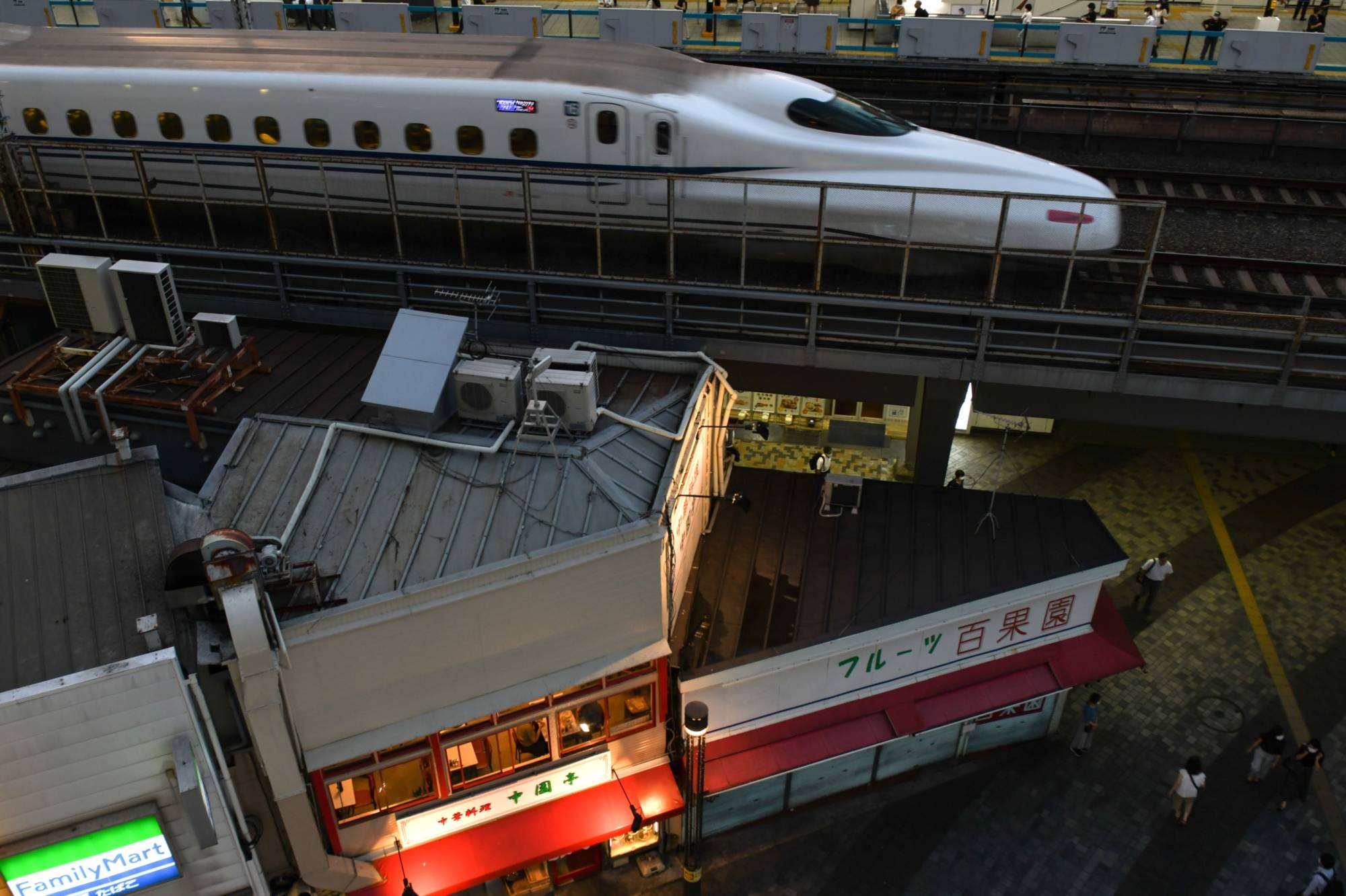An aerial image provides a detailed view of an urban setting featuring a bustling scene below. Centrally, a restaurant with a white exterior and distinctive red awnings stands out prominently. Signs on the building bear Chinese or Japanese text, further emphasizing its ethnic theme. Surrounding the restaurant are a few smaller shops, one with a blurred green sign, and a noticeable number of people—about 10 to 20 in total—scattered about, including some alongside a railing near the restaurant. The street below appears to be cobblestone, adding texture to the scene. Above this, towards the upper part of the image, an elevated railway track cuts across from left to right, where a sleek bullet train, white with blue stripes and multiple windows, glides along. The train's metallic sheen and pointed front contrast with the urban landscape, making it a significant focal point of the photograph.